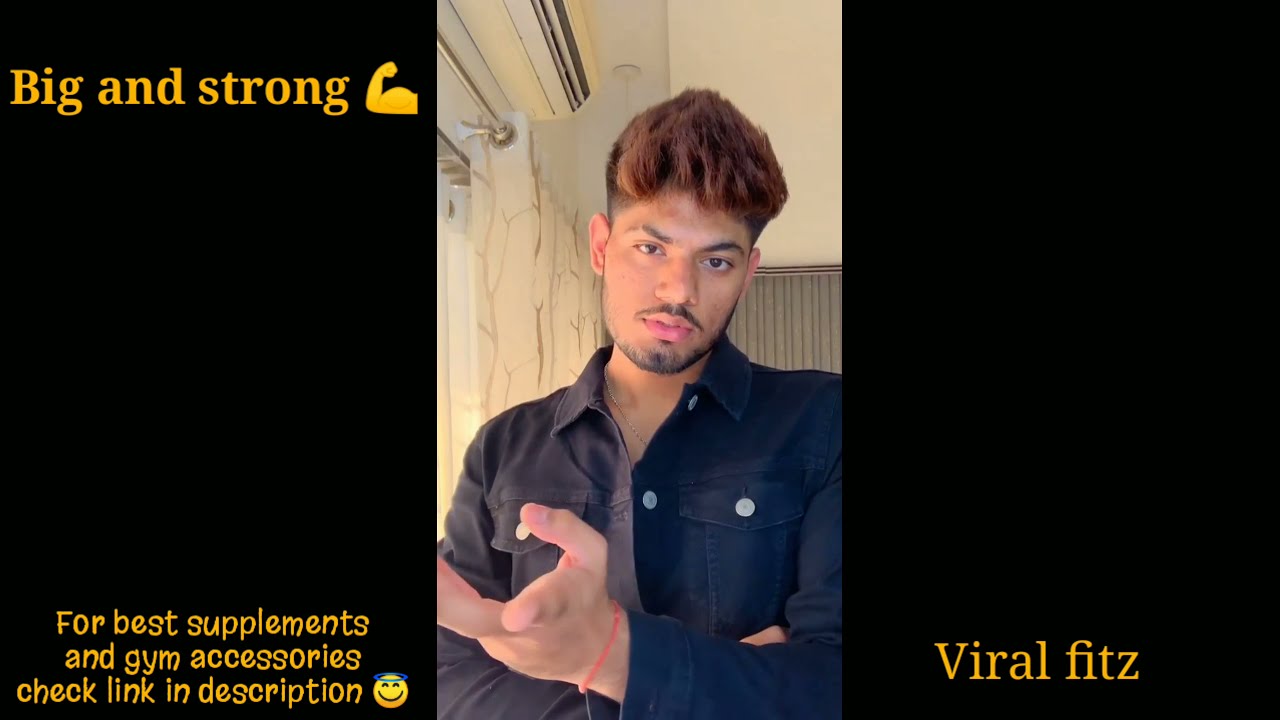This is an advertisement for fitness supplements and gym accessories. The central figure is a young man of apparent Indian heritage, possibly in his mid-twenties to early thirties, with brown skin, dark spiky hair with a deep brown top, black eyebrows, a mustache, scruffy beard along his neckline, and dark brown eyes. He has full lips and a broad nose. He is dressed in a blue or black denim-like buttoned-up jacket with silver buttons, accentuated by a thin orange or red bracelet around his left wrist. His left hand is making a gesture as if explaining something to the viewer. 

The background appears to be an apartment setting, featuring an air conditioner to the top left and a curtain behind him. On both left and right sides of the image are large, black wide bands. The left band displays the bold yellow-orange text "BIG AND STRONG" with a flexed bicep emoji below it. Underneath in smaller letters, it reads, "For best supplements and gym accessories, check link in description," punctuated with a smiley face with a halo. The right band contains the text "VIRALFITZ" in gold letters at the very bottom.

This comprehensive and detailed view presents the young man in a setting that reflects the theme of fitness and strength, complemented by clear and promotional messaging on either side.